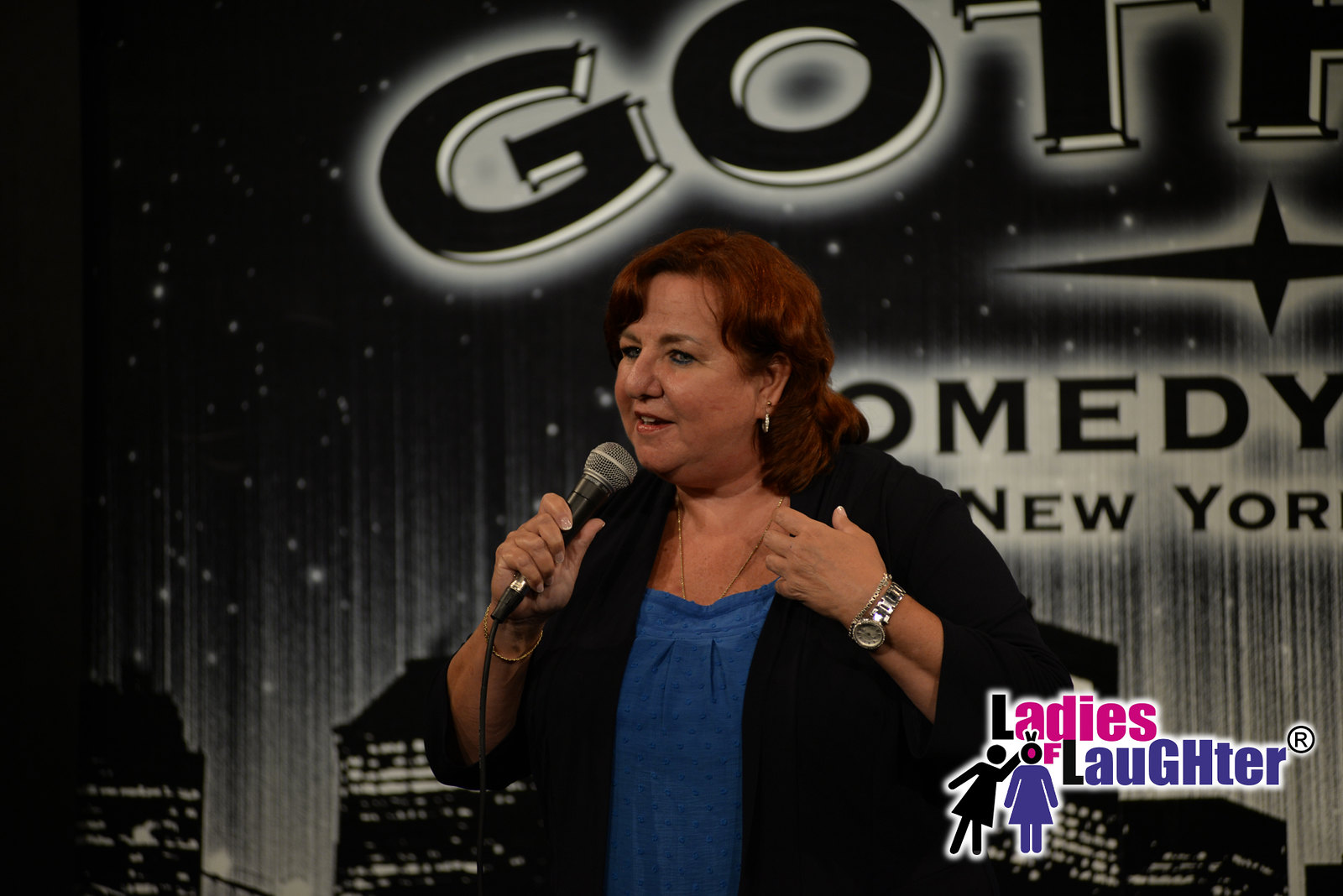The image depicts an indoor setting at what appears to be a comedy club, with a middle-aged woman standing center stage. She has medium-length reddish hair and is wearing silver hoop earrings. Dressed in a black jacket over a blue top, she accessorizes with a silver-tone watch and a necklace. She is holding a microphone, which suggests she is a stand-up comedian. Notable details include her long shiny fingernails and a golden bracelet. The backdrop features a black-and-white graphic with a partially visible text that reads "GOT" and "Comedy New York," accompanied by an image of buildings and stars. In the bottom right corner, there is a logo for "Ladies of Laughter," featuring two icons of women—one in black and the other in purple—with the text in black, pink, and purple colors.